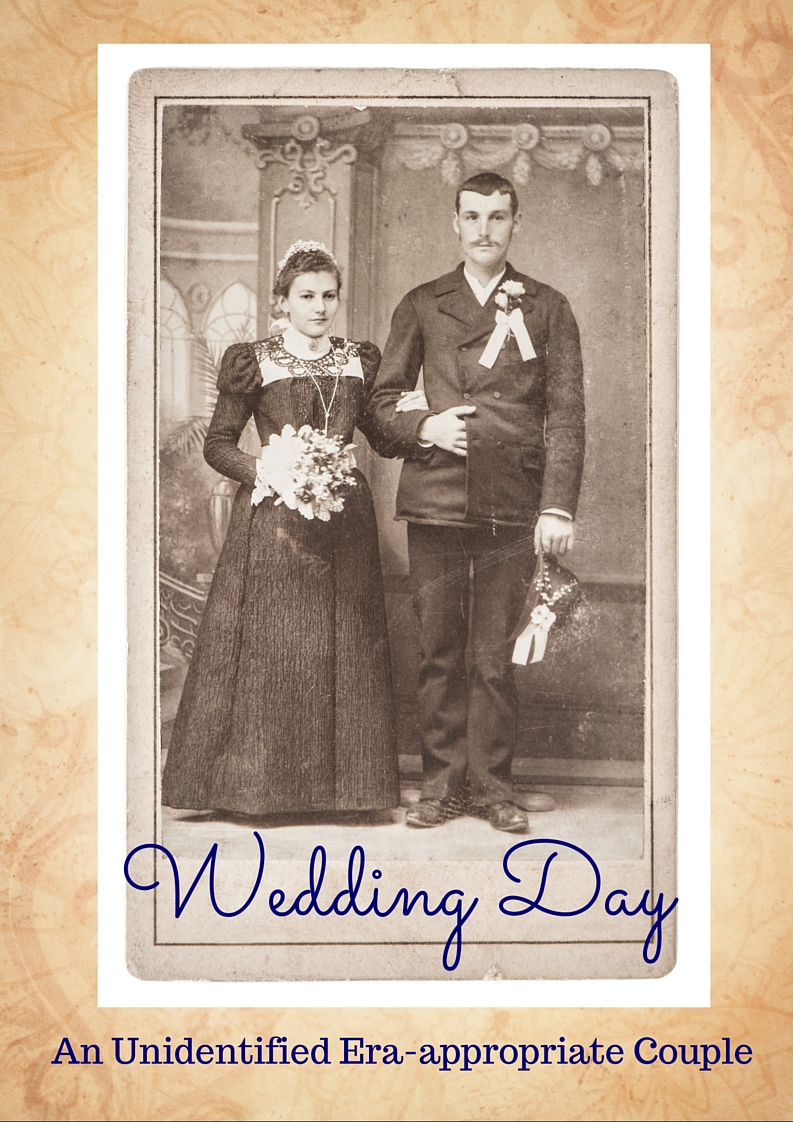In the image, there is an old, faded black-and-white picture of a couple standing next to each other, reminiscent of a photo frame with light brown, ornate borders. On the right stands a very tall Caucasian man with short brown hair, dressed in a dark brown suit buttoned up to the neck. His right hand, holding a handkerchief, rests by his hip, while his left hand is curled inside his suit jacket just in front of his stomach. Next to him is a woman whose head reaches up to his neck. She is wearing a long black dress and holding a bouquet of flowers in front of her stomach. She has dark brown hair adorned with a white display on top. At the very bottom of the photograph, "Wedding Day" is written in dark blue cursive text. Surrounding the entire photo is a white square frame, backed by an orange background, with additional purple text at the bottom reading, "An Unidentified Era Appropriate Couple."